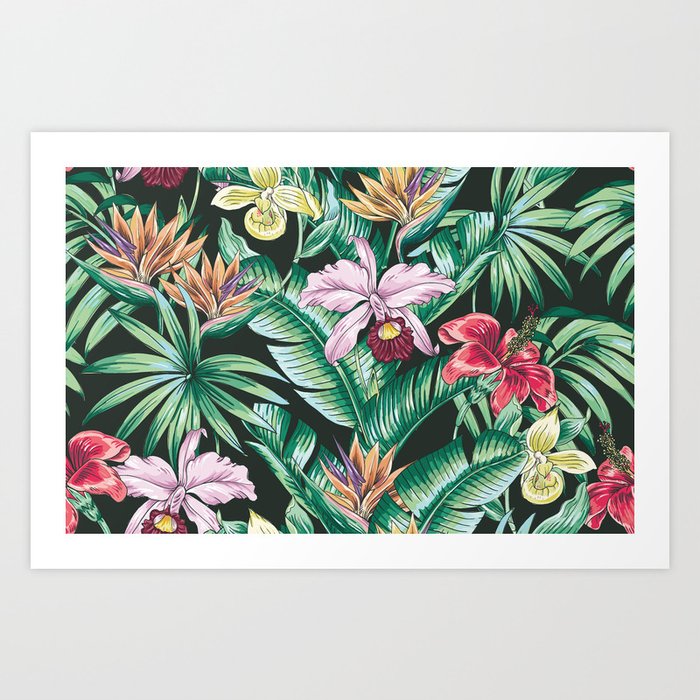This detailed artistic photograph captures a vibrant composition of tropical flora against a striking black gradient background. The image, styled akin to a product showcase for wall art, features a rectangular canvas with a thick white border, giving it an elegant presentation. Predominantly, the scene is filled with an array of green foliage, including dark green palm fronds and wide, fern-like leaves, drawn with colored pencils to give a realistic touch.

Scattered throughout the lush greenery are multiple types of vividly colored flowers: red hibiscuses with yellow centers, yellow daffodils, and orange and purple birds of paradise. Light pink flowers with dark red centers and a touch of yellow also add to the scene’s diversity. Positioned meticulously are groups of flowers, such as red, orange, pink, and yellow ones, creating a harmonious blend of colors. Notably, the flowers in the bottom left corner are red with yellow or pink petals, while the top left section displays yellowy-orange blooms. The central top features yellow and orange flowers, just below which are pink flowers. Near the bottom right corner are more red flowers, accompanied by yellow ones.

In total, this intricate display includes approximately 12 to 15 different floral elements, all interconnected by lush green leaves, presenting a vivid and detailed depiction of tropical nature.